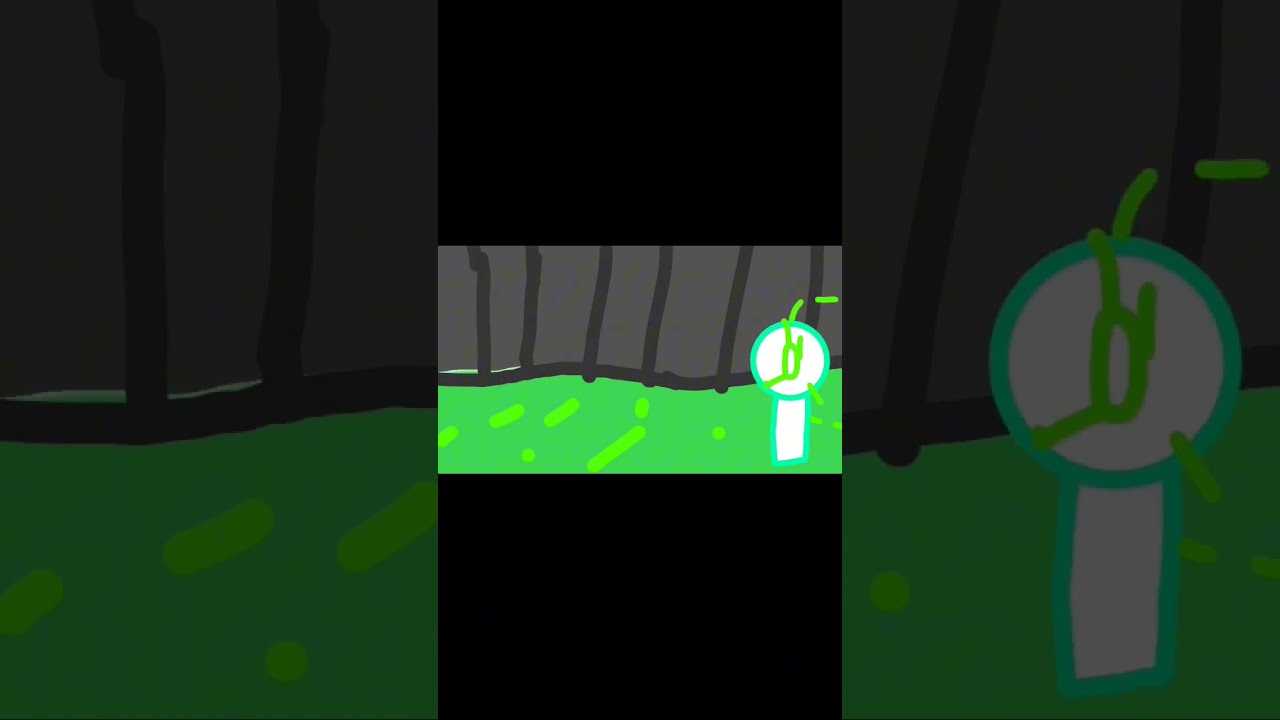The image is a digital drawing with a central landscape-oriented frame superimposed on a larger canvas. The central portion of the image is flanked by black rectangular bars above and below, with the middle section featuring a digital artwork. This artwork depicts a division between a vivid, bright green grass area on the bottom and a dark brown or gray fence with vertical lines that bend and appear crooked in certain places. The background behind the fence is a uniform gray.

Towards the right side of the image, there is a notable figure resembling a sign. This figure consists of a white rectangle at the bottom with a white circle on top, outlined in aqua green or light blue. Inside the circle, there's a symbol resembling an eye with dashed lines or an antenna extending from it. The green grass at the bottom is interspersed with lighter green shapes, including circles and elongated forms. This central visual is mirrored and darkened on both the far left and far right edges of the entire composition, creating a repetitive and balanced effect.